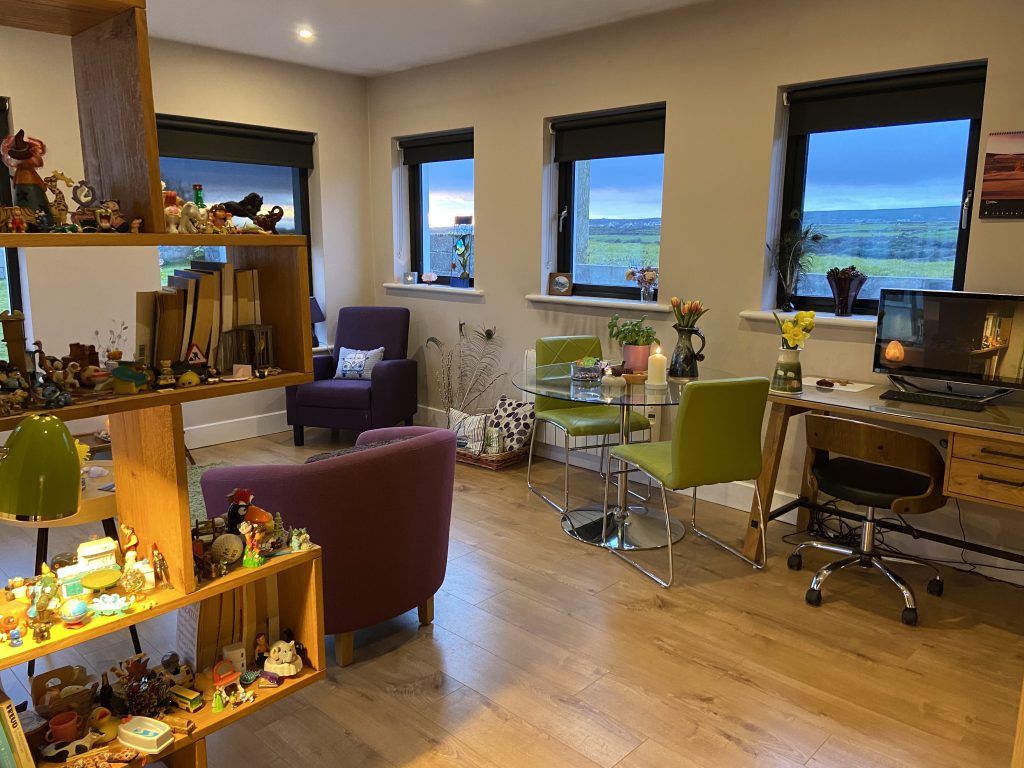The image portrays a well-lit indoor living space with a mix of modern and eclectic decor. Four square windows with rolled-up black shades line one wall, revealing a flat, grassy landscape outside under a cloudy sky. The windowsills are adorned with various plants, knick-knacks, and a Galileo thermometer in the farthest window. To the right of the image, there's a brown wood desk with a glass top, accompanied by a rolling chair and two drawers. A computer monitor sits on the desk next to a vase of yellow flowers. Nearby, a glass table with a chrome pedestal base is surrounded by two green, armless, padded chairs with metal legs. In the foreground, freestanding open-back cubby shelves house an array of doodads, figurines, books, and a lamp with a green shade. A decorative basket with floor pillows and some large peacock feathers is placed behind the table. The seating arrangement includes a navy blue chair with a VW bus throw pillow in the far corner, a purple club chair with wooden feet facing left, and additional colorful fabric seats scattered throughout. The room exudes a cozy, lived-in atmosphere, possibly functioning as a home office or waiting area.